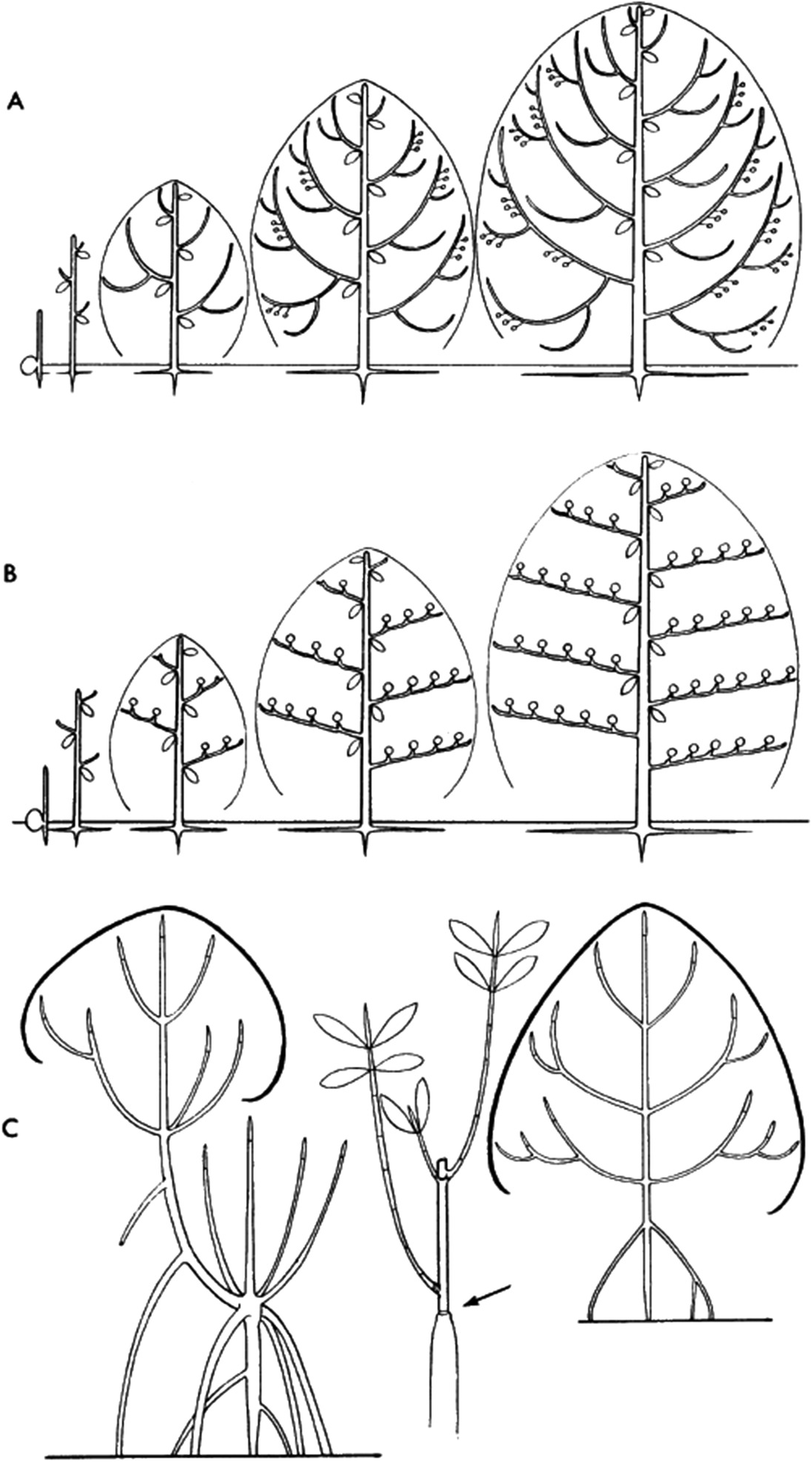The image is a black and white textbook drawing depicting the growth stages of three different plants, labeled A, B, and C from top to bottom. Each set of diagrams shows the development of a plant from a simple stem to a fully grown structure. 

- **Diagram A:** Starting on the left, the sequence begins with a basic stem, which gradually grows larger and develops multiple branches and leaves, eventually forming a fully mature bush. 
- **Diagram B:** Similar to A, this sequence illustrates a plant's growth from a stem with a few leaves to a fully developed plant, differing mainly in its simpler design and the addition of more leaves on the stems.
- **Diagram C:** This set is more complex and depicts a plant that grows multiple stems from the ground, which then conjoin and form various branches. It has a less straightforward pattern compared to the others, with branches extending in multiple directions.

Overall, the image effectively illustrates the progression of plant growth in three distinct styles.